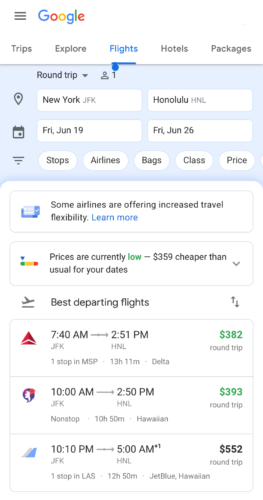The image captures the screen of a smartphone displaying a Google search page dedicated to flight planning. At the top is the iconic multicolored Google logo. Below it are tabs labeled "Trips," "Explore," "Flights," "Hotels," and "Packages." The search query indicates a round trip from New York's JFK Airport to Honolulu, Hawaii, scheduled from Friday, June 19th to Friday, June 26th.

The top section of the screen is highlighted with a blue background, featuring details such as the number of travelers (1) and options for stops, airlines, baggage, class, and price filters. Below this section, the screen transitions to a white background with a message stating, "Some airlines are offering increased travel flexibility, learn more." It also notes that current prices are $359 cheaper than usual for the selected dates.

Scrolling down further, one can see a section titled "Best departing flights," showcasing a list of flight options. Each entry includes icons on the left, departure and arrival times, number of stops, total flight duration, and specific airlines like Delta, Hawaiian, and JetBlue. The prices for these flights are displayed in green, with options ranging from $382 and $393 to $552.